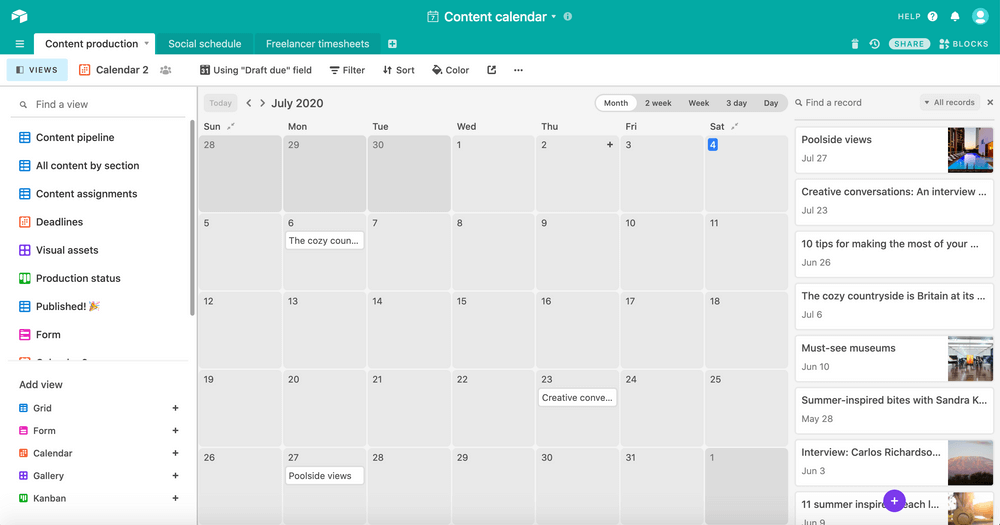The horizontally rectangular image is a detailed screenshot from a calendar app interface, framed with a teal green horizontal banner at the top, centrally labeled "Content Calendar." On the left side of the banner, three tabs are visible: "Content Production," "Social Schedule," and "Freelancer Time Sheets," with the "Content Production" tab currently selected. 

Beneath these tabs is a vertical listing of content management categories: "Content Pipeline," "All Content by Section," "Content Assignments," "Deadlines," "Visual Assets," "Production Status," "Published," "Form." At the bottom of this listing is a feature labeled "Add View" offering options such as "Grid," "Form," "Calendar," "Gallery," and "Kanban."

To the right side of the image is a vertical column showcasing various scheduled content items with their respective dates. The entries include:
- "Poolside Views" scheduled for July 27th,
- "Creative Conversations" on July 23rd,
- An entry starting with "10 Tips for Making the Most of Your..." with titles cut off, dated June 26th,
- "The Cozy Countryside is Britain at its..." dated July 6th,
- "Must See Museums" on June 10th,
- "Summer Inspired Bites with Sandra" slated for May 28th,
- "Interview Carlos Richardson" scheduled for June 7th.

The central portion of the image is occupied by a calendar display set to July 2020, bridging the two columns and providing a structured overview of content scheduling.